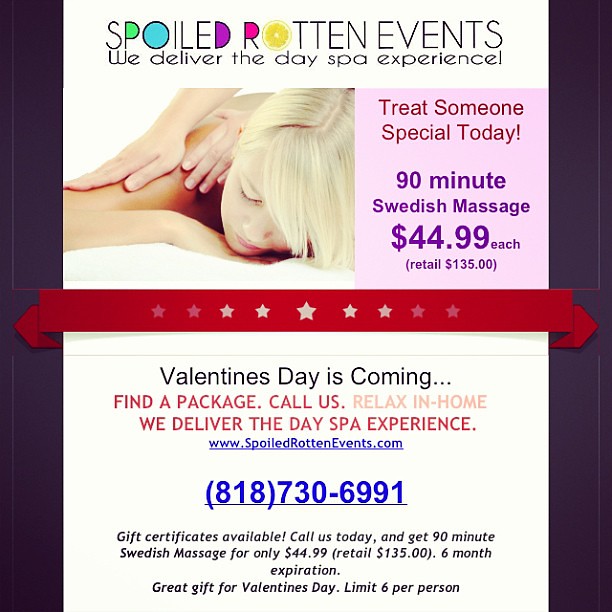The image is an advertisement for Spoiled Rotten Events, prominently featuring bold, colorful text set against a purplish background. It announces, "Spoiled Rotten Events" at the top in vibrant letters, including green, blue, purple, magenta, and an orange "O" in "rotten". A red ribbon with white stars fading to red at the edges stretches across the center. The main text reads, "We deliver the day spa experience. Treat someone special today. 90 minute Swedish massage, $44.99 each (retail $1.35)." It emphasizes the upcoming Valentine's Day with a call to action: "Valentine's Day is coming. Find a package. Call us. Relax in home. We deliver the day spa experience. Gift certificates available." On the left side, an image shows a person receiving a massage. The advertisement borders are black, framing the colorful display. Contact details include a phone number (818-730-6991) and a website (spoiledrottenevents.com). The text varies in colors such as black, red, purple, and blue, making the flyer eye-catching but slightly chaotic in design.